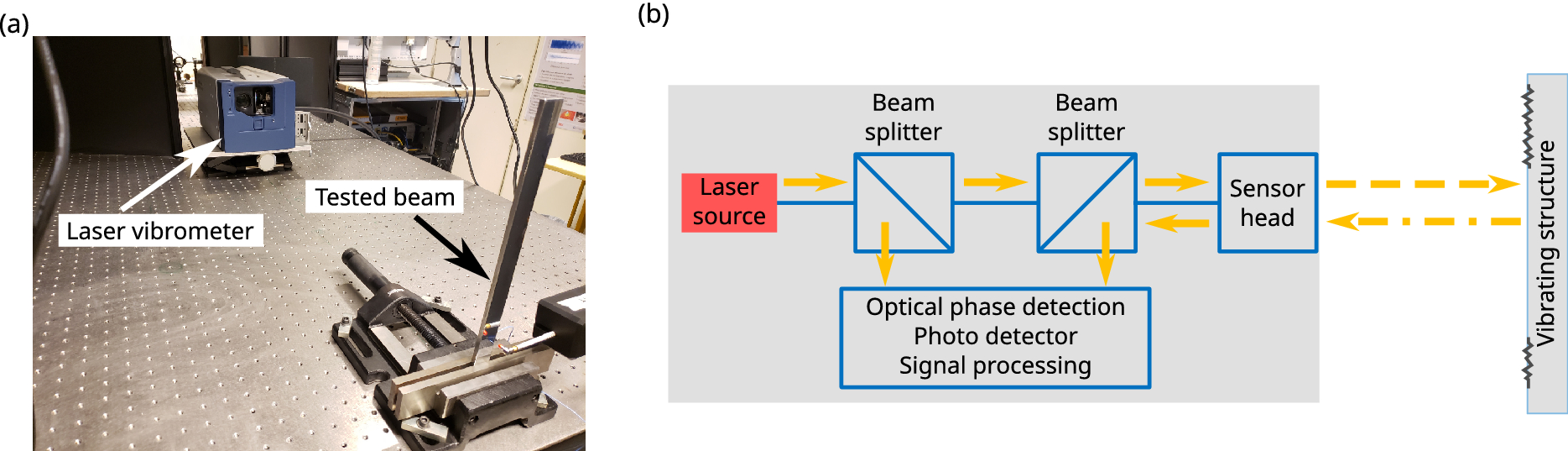The image is arranged in a landscape orientation, divided into two distinct sections labeled "(a)" and "(b)." 

- **Section (a):** This is a photograph depicting a lab setup. At the top of this section, there is a label "(a)" followed by a small square image of a lab table. This table is silver and has several holes in it. On the table, there is a blue box identified as a "laser vibrometer," denoted by a white rectangle with black lettering. An arrow points from the label to the blue box. Adjacent to this, a tall L-shaped metal beam stands vertically on its short side, labeled "tested beam" with a black arrow pointing towards it.

- **Section (b):** This section features a detailed diagram with the label "(b)" at the top. The diagram starts with a small red box labeled "laser source" on the left side. From the laser source, a blue line extends to a diagonally split blue box marked "beam splitter," with a yellow arrow following the path. The beam splitter directs the laser beam downwards with another yellow arrow to a second blue box labeled "optical phase detection, photo detector, signal processing." Simultaneously, a secondary beam is directed from the beam splitter to another sensor head depicted as a blue box with a corresponding yellow arrow. All these components are connected by a dashed line to a separate vertical gray box on the right side, labeled "vibrating structure," which includes gray squiggly lines to signify vibration.

This composite image effectively contrasts a physical lab setup with its corresponding functional diagram, detailing the elements involved in laser vibrometry and beam testing.